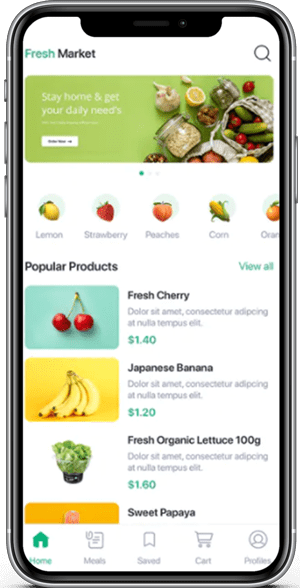This image is a screenshot of a smartphone displaying a grocery shopping app named "Fresh Market." At the top of the screen, the app's name is stylized with "Fresh" in green and "Market" in gray. Adjacent to the name is a gray magnifying glass icon, signifying a search function. The screen features a headline that reads, "Stay home and get your daily needs," set against a green backdrop adorned with colorful images of various foods. The vibrant array includes red and green peppers, other assorted vegetables, and a lemon, all packed in bags and jars.

Below the headline, there is a selection of categorized food options. Each category is represented with an icon: a lemon icon paired with the word "Lemon," a red and green strawberry icon next to "Strawberry," an orange and green peach icon with the label "Peaches" in gray text, and a yellow and green corn icon beside the word "Corn."

The section labeled "Popular Products" showcases images and names of frequently bought items: "Fresh Cherry" with an image of a red cherry, "Japanese Banana" featuring a prominently yellow banana against a yellow background, and "Fresh Organic Lettuce 100g," which shows green lettuce in a silver container.

At the bottom of the screen, there is a navigation bar with icons and labels for different sections: Home, Meals, Saved, Cart, and Profile. The majority of the background is white, complementing a variety of food images that add both vibrancy and context to the app’s user interface.